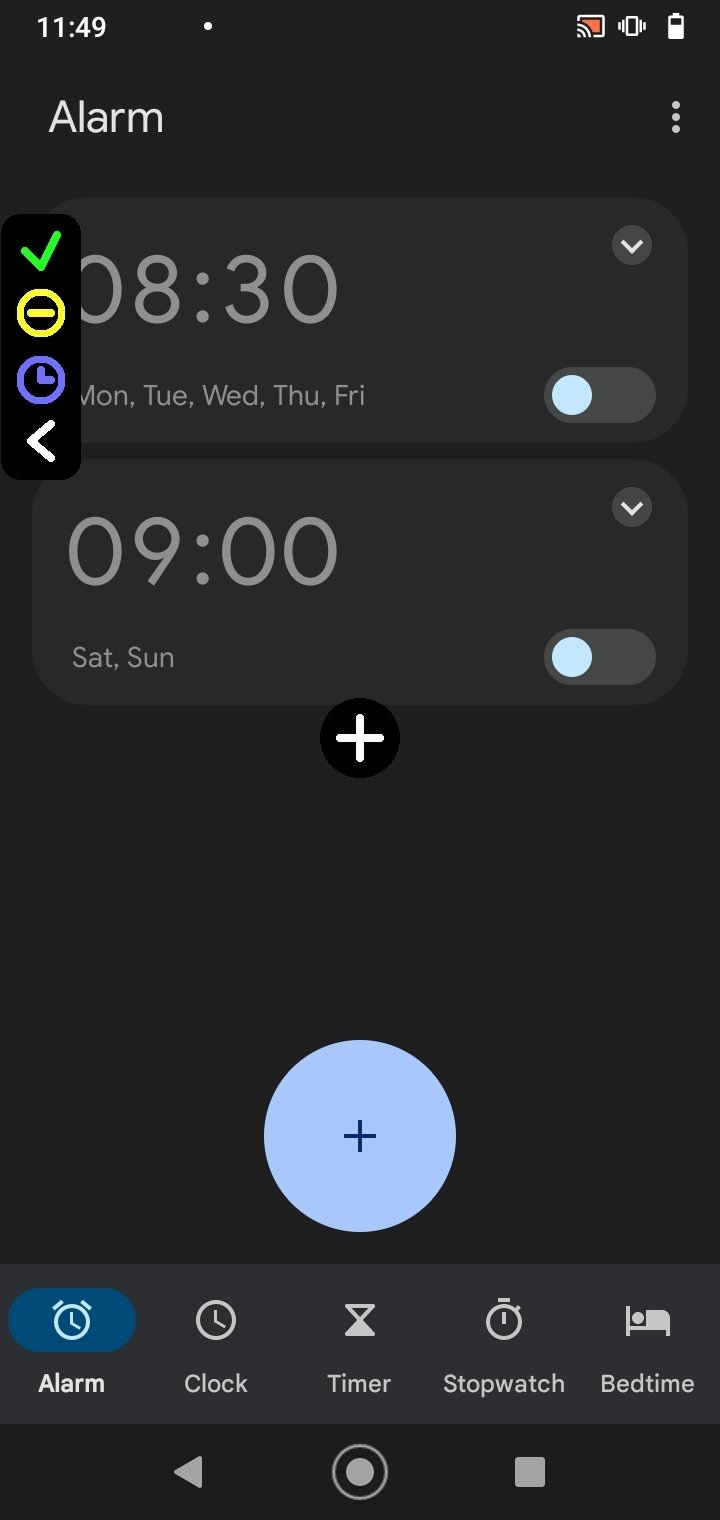The screenshot is taken from a cell phone displaying the alarm clock settings page. The background is black, and the current time shown in the top left corner is 11:49. On the top right, the status bar displays the battery level and a small lock icon, indicating the screen is locked.

Below the time, the word "Alarm" is prominently displayed to indicate the section of the app being viewed. To the right of the word "Alarm," there are three vertical white dots, typically signifying a menu or additional options.

In the upper half of the image, there is a gray rectangle displaying the alarm time set for 08:30, along with the days it is scheduled to repeat: Monday, Tuesday, Wednesday, Thursday, and Friday. Adjacent to this is an on-off switch, which appears to be set to off, as indicated by the switch being positioned to the left.

Below this first alarm, there is another gray rectangle showing another alarm set for 09:00, with the days Saturday and Sunday listed. Similarly, this alarm also has an on-off switch that is currently set to off.

In the center of the image, there's a smaller black circle containing a white plus sign, likely for adding new alarms.

Near the bottom, there is a large blue circle with a black plus sign inside it, indicating an option to add a new alarm as well. Beneath this, a navigation bar is visible with different icons and options. The active section is "Alarm," as shown by the blue oval highlighting the alarm clock icon. Other options in this bar include "Clock," "Timer," "Stopwatch," and "Bedtime."

Overall, the screenshot meticulously details the alarm settings and options available on the user's cell phone.